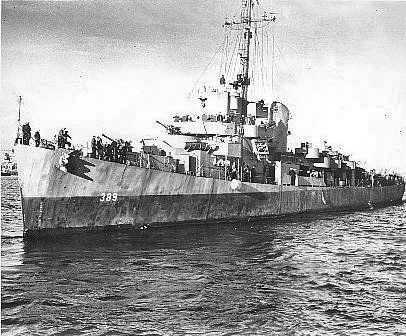A grainy black-and-white photograph depicts a mid-sized United States Navy destroyer at sea, likely from World War II. The image shows a three-quarter view of the ship's port side, with the hull number “389” prominently displayed on the bow. The vessel features a two-tone paint scheme, with a darker gray bottom half and a lighter gray upper half. The destroyer is equipped with multiple gun turrets and torpedo racks, all appearing to point forward, along with a single funnel and a central mast behind the bridge. Sailors can be seen standing on deck, although the graininess of the photograph makes them appear hazy. The destroyer is surrounded by still, dark water, and the faint outline of other ships can be seen in the background, suggesting proximity to a port. The overall composition includes the ocean and a light sky, painting a solemn scene of naval strength.